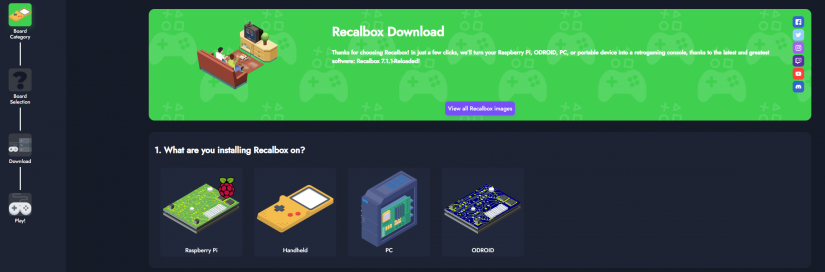**Caption:**

The image appears to be a promotional graphic for a "Recall Box" download, meticulously showcasing various visual elements reminiscent of the popular game Minecraft. The primary focus is a central, green-colored box, depicting a group of people enthusiastically engaged in a video game, with an Xbox controller wallpaper adorned in the background. Above the green box is a header with the misspelled word "recall" (spelled with only one 'l').

Beneath this box, centrally in blue text, is the phrase "View All Recall Box Images." To the right, social media icons for platforms like Facebook, Twitter, and YouTube are prominently displayed.

Under the main image, there is instructional text reading, "Number 1: What are you installing a Recall Box on? You can do it on the Pi, a handheld, a PC, or an Odroid.” Each option is represented by images such as the Raspberry Pi, indicating its computer system designed for video game emulators. 

On the left column, labeled as the board category, a similar image of a handheld device within a green box is shown. Adjacent icons include a board selection with a question mark, a download icon with a controller, and a play button, connected by lines to illustrate the sequential steps for using the Recall Box. The background features a brown rug and a TV set atop a cabinet, adding to the cozy, home-gaming atmosphere depicted in the graphic.